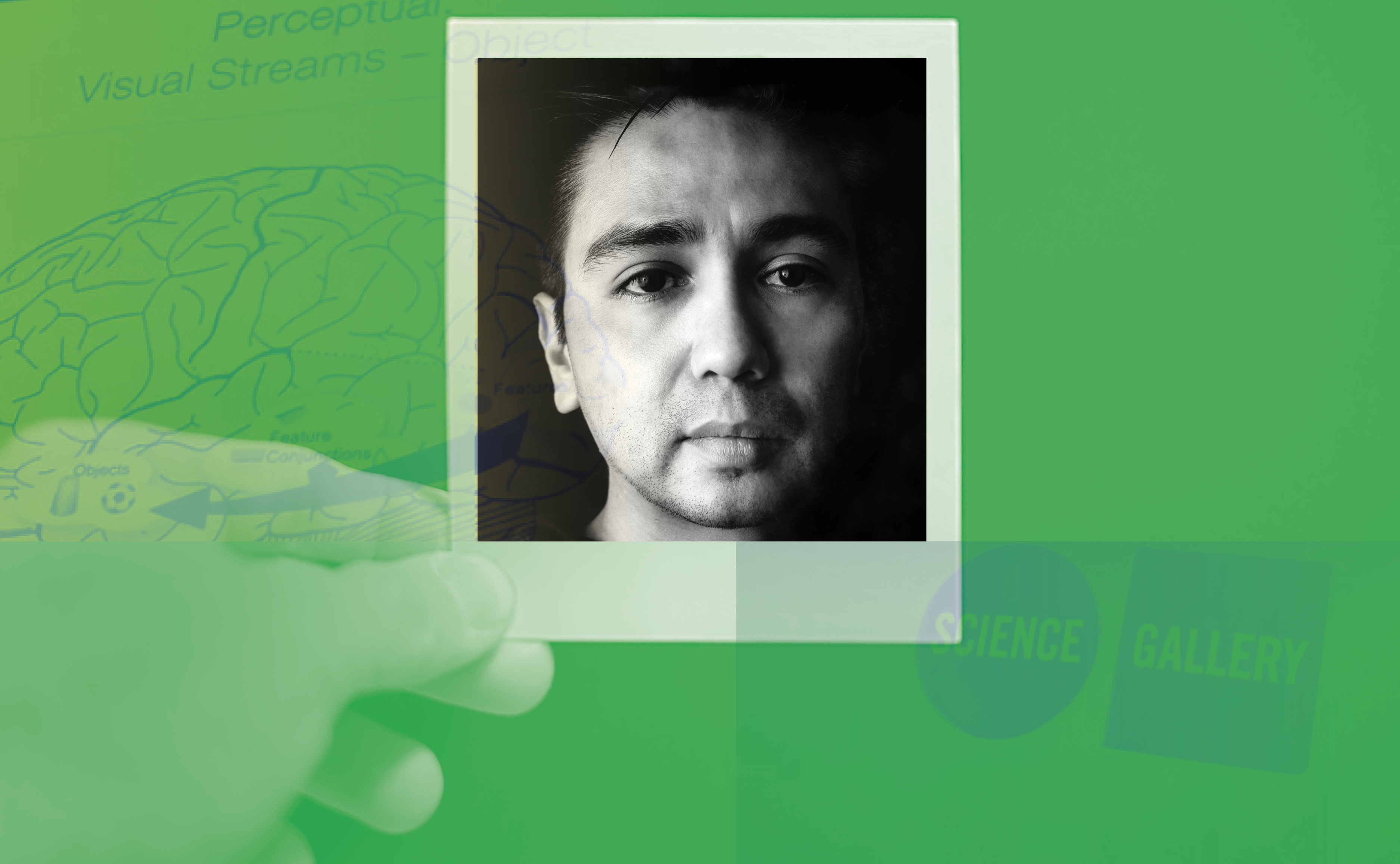In this striking and complex graphic, the focal point is a black-and-white Polaroid photograph of a man with fair skin, dark eyes, and black hair. His expression is serious and somewhat sad, as he gazes just past the camera. The Polaroid is being held by a semi-transparent hand, gripping it by the lower left-hand corner. The background of the graphic is predominantly green, displaying faint, ghostly images of a brain and various overlaid words. Among these barely visible text elements are "perception," "visual streams," "science," and "gallery." An arrow extends outward from the brain image, adding an additional layer of scientific intrigue and complexity to the composition. The man's face is illuminated from the left side, creating a dynamic interplay of light and shadow. Overall, the graphic merges elements of human emotion with scientific motifs, offering a visually arresting and thought-provoking scene.